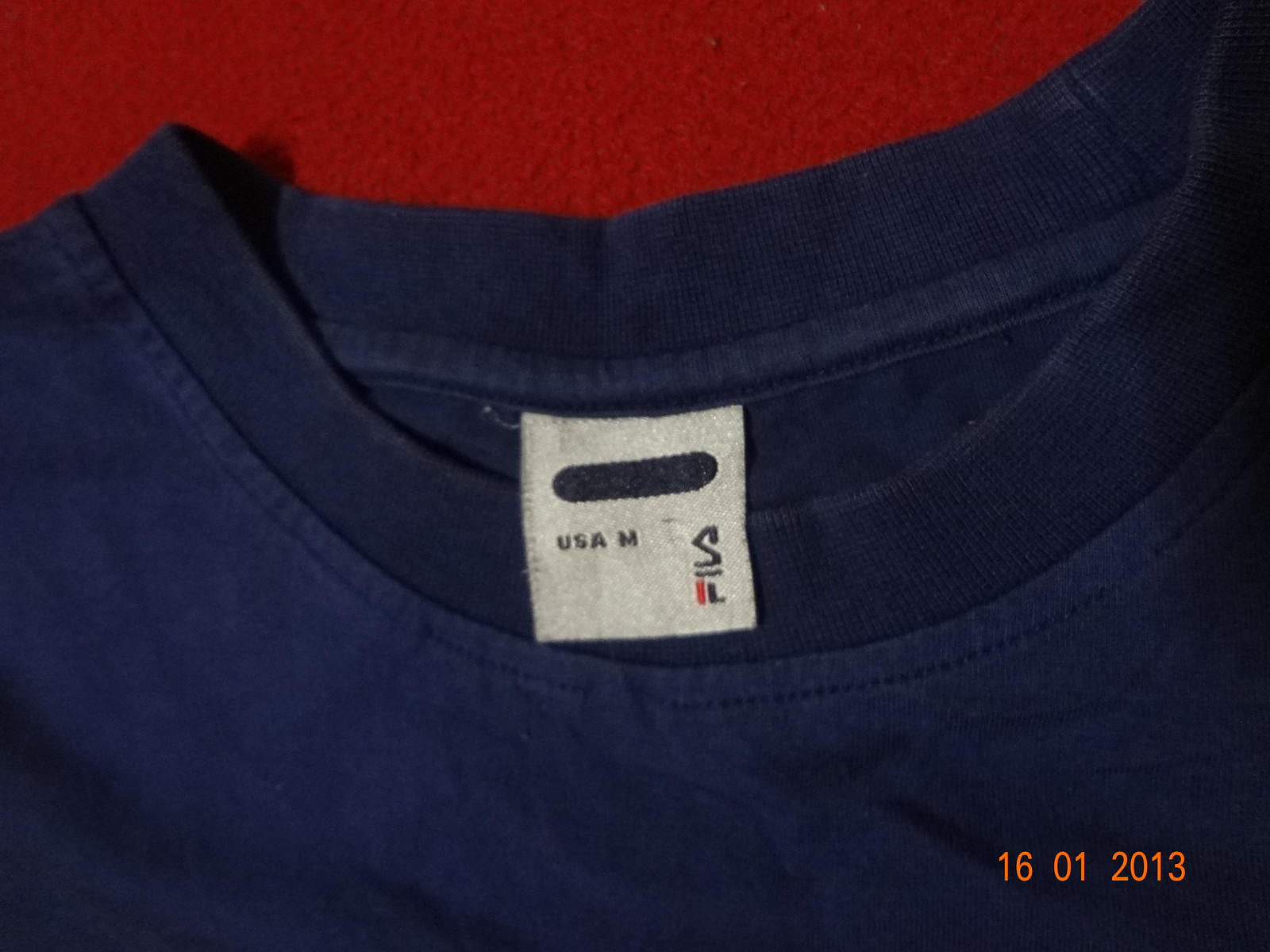A close-up image captures the upper region of a t-shirt collar, spanning from the center-top to near the top-right corner. The shirt is laid out on a red cloth that provides a stark contrast to its fabric. A white tag is visible on the back of the collar, with an elongated black oval flanking each side. The tag features the text "USA" along with a medium size designation and a small black "M" printed at the end.